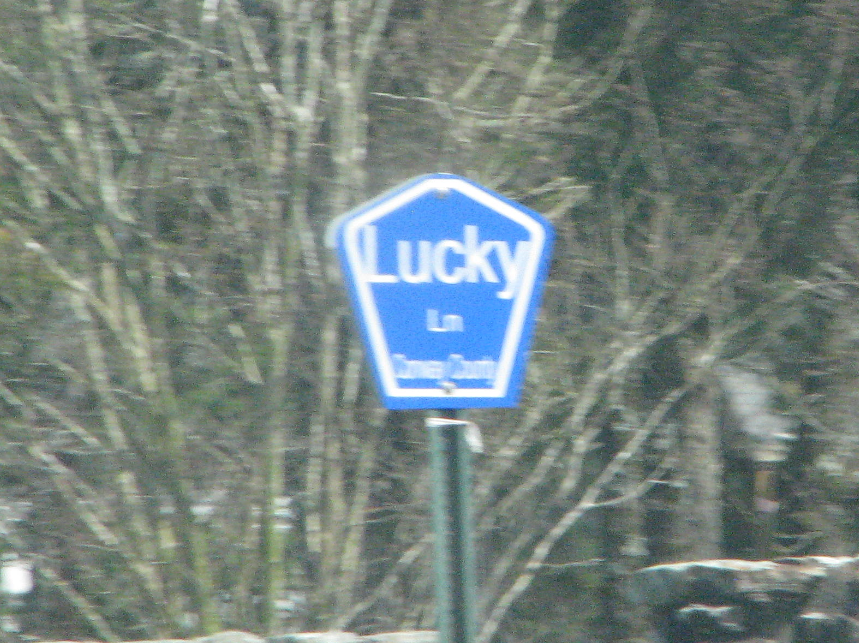This daytime photograph, taken outdoors, captures a dark blue, five-pointed, trapezoidal sign featuring a white outline and bold white text. The sign prominently reads "Lucky Lane" in clear letters, with additional, blurred text below that appears to mention "County." The sign is mounted on a dark green pole, about a foot and a half visible in the frame. The background consists of mostly leafless, thin, and stark branches, suggesting a winter setting, with some green foliage scattered throughout. There are also stone-lined walls to the right and faint outlines of buildings and trees with dark brown trunks. The image is somewhat grainy and blurry, potentially showing patches of white snow on the ground.